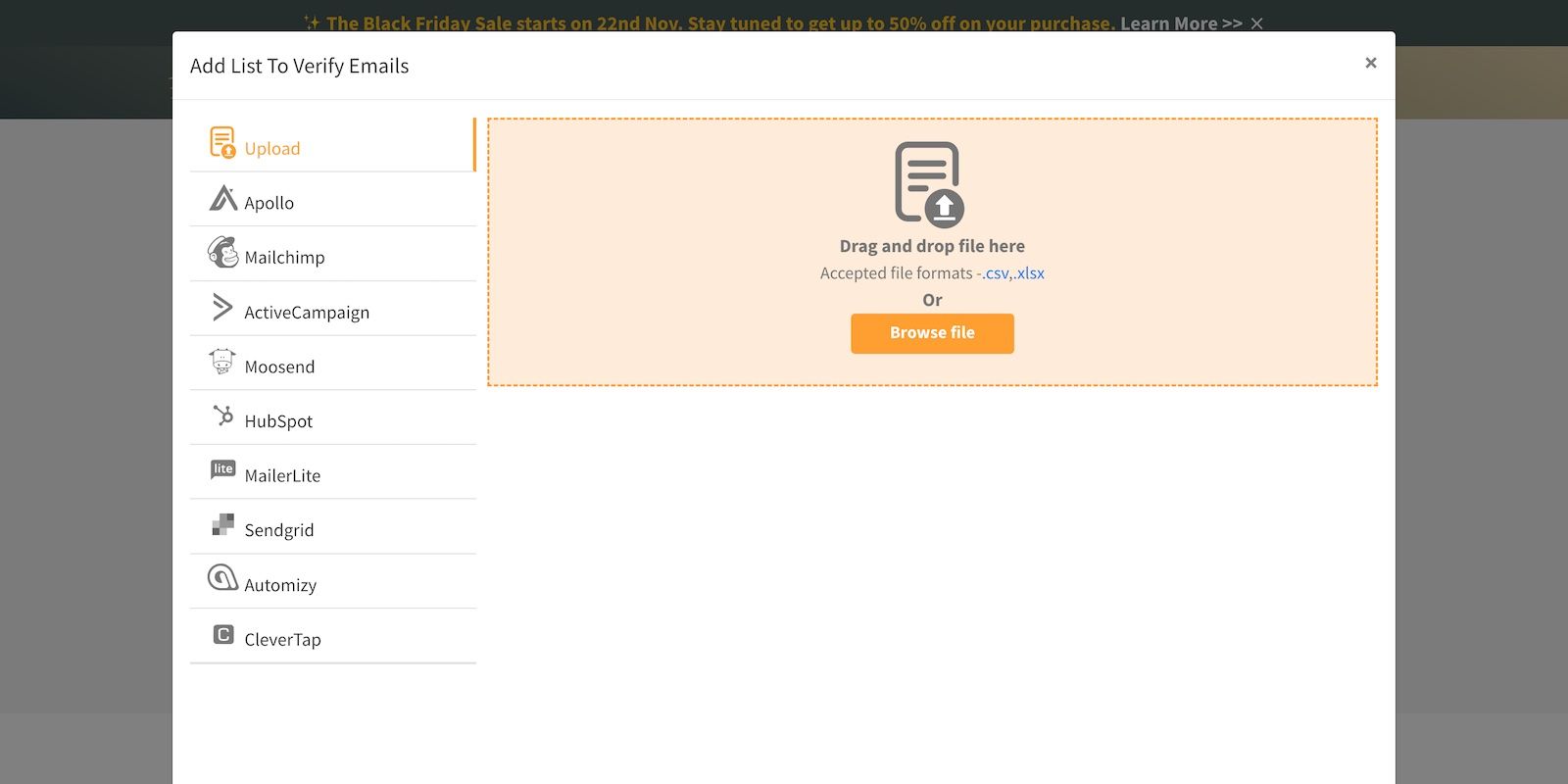This is a detailed screenshot of a website featuring a prominent white pop-up menu that obscures the majority of the website behind it. At the top of the website, there's a black bar with faint text announcing, "Black Friday sale starts on 22nd November. Stay tuned to get 50% off your purchase. Learn more."

The white pop-up menu dominates the center of the screen. At its top, the menu prompts users to "Add list to verify emails," and to the right, there's a small 'X' for closing the menu. Below the title, there is a vertical list on the left side with various choices, including:

1. Upload (selected with a yellow highlight),
2. Apollo,
3. MailChimp,
4. ActiveCampaign,
5. MooseEnd,
6. HubSpot,
7. MailerLite,
8. SendGrip,
9. Automacy,
10. Clevertap.

When "Upload" is selected, it turns yellow, and the right section of the menu changes to an upload interface. This section is a large pale orange rectangle featuring a centered gray icon of a page of paper with a white arrow pointing upwards inside a circle at the lower right. Below the icon, the gray text directs users to "drag and drop file here."